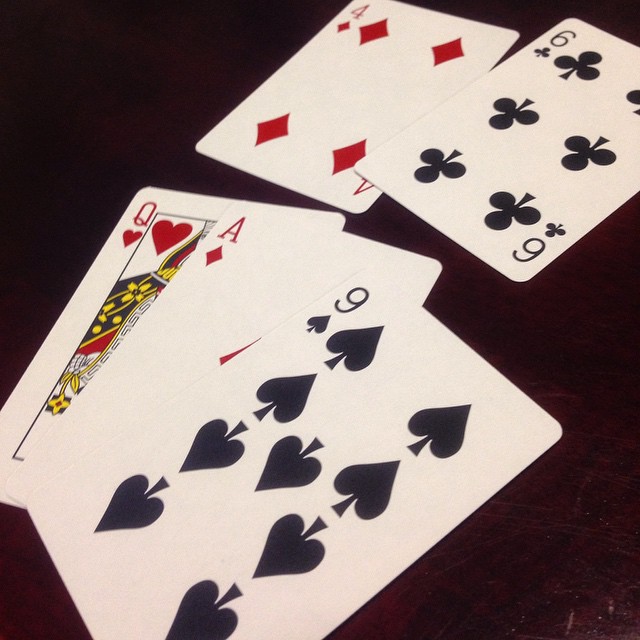The image features five face-up playing cards arranged against a solid black background. The layout consists of two cards at the top and three at the bottom. The upper two cards, which slightly overlap each other, are the red Four of Diamonds and the black Six of Clubs. Below them, three cards overlap considerably but remain identifiable: the red Queen of Hearts, the red Ace of Diamonds, and the black Nine of Spades. The careful arrangement allows each card's value and suit to be visible despite the overlapping.